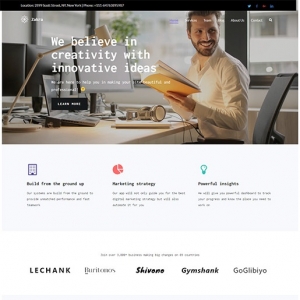The webpage features a vibrant and detailed layout with several elements. Dominating the page is an image of a person smiling and gazing to the right, dressed in a white dress shirt paired with black pants. The individual has a completely shaved beard and mustache, with brown hair, and is holding an open book. The book's binder is a striking combination of orange and tan, contrasting with its white pages.

To the left of this image, bold white text reads, "We believe in creativity with innovative ideas." Additional smaller white text, though hard to discern, accompanies this statement. Below the text sits a rectangular black button inscribed with the words "Learn More" in white.

Located to the person's right is a diverse array of equipment, which includes silver and gray headphones with distinctive white circles and a gray laptop. Behind this setup, windows reveal a backdrop of green leafy trees. A bending light fixture with a cylindrical white top is also noticeable.

At the bottom of the section, a purple building is highlighted with black text stating, "Build from the ground up." Accompanying this are various graphical elements: a fragmented red pie chart labeled "Marketing Strategies" in black, and a teal light bulb icon with the phrase "Powerful Logistics" in black.

Underneath these components are names and words associated with different businesses or entities. One prominent name is "LECHANK" in bold black text. Following it is another name obscured by blurriness. Also, in bold black, are the names "SHIVOMO," "Gymshark," and another somewhat unreadable name seemingly spelled "GOGLIBIYO."